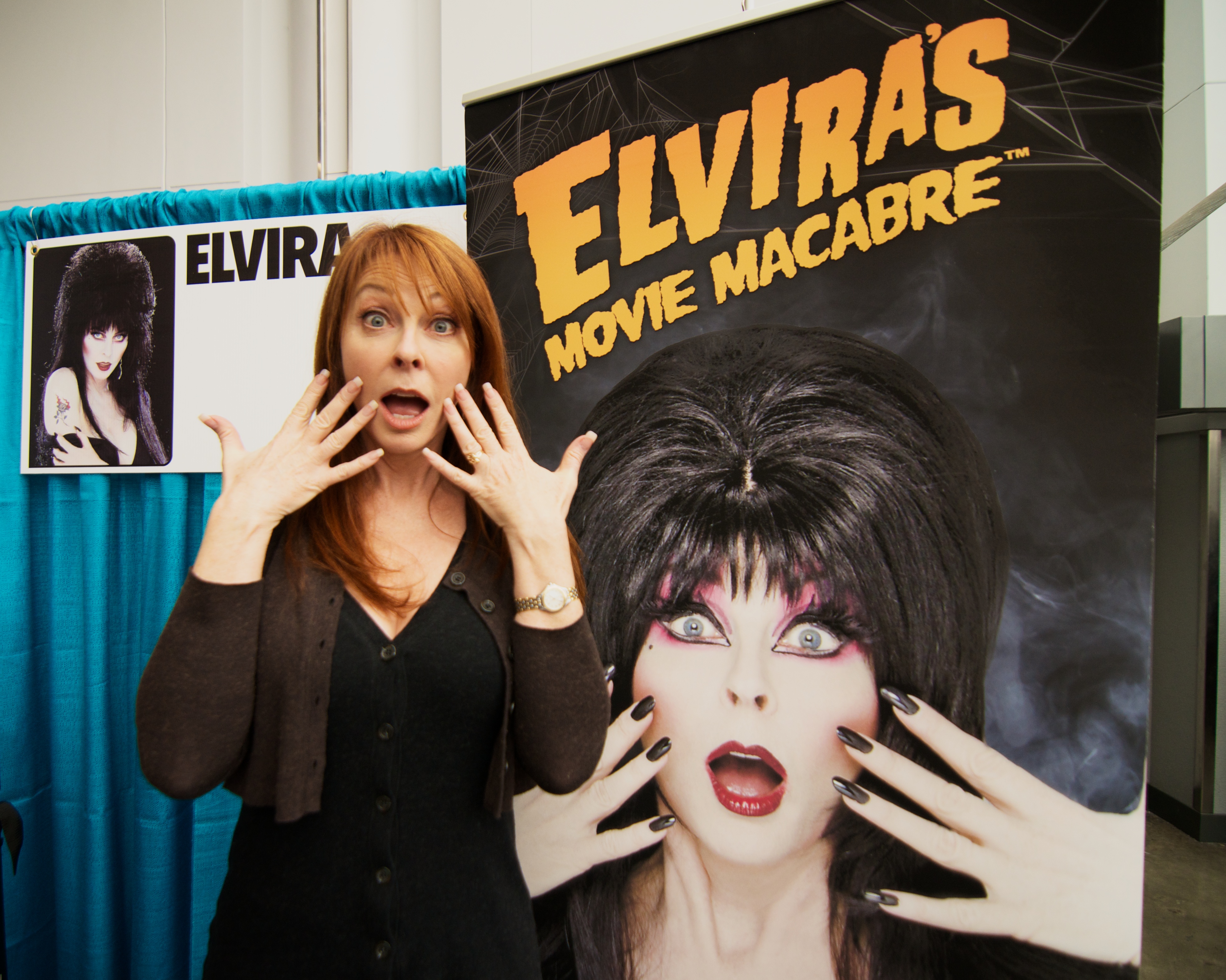In this indoor photographic image, we see the actress who portrays Elvira, a famous horror movie character, standing in front of a promotional backdrop for "Elvira's Movie Macabre." The actress, a white woman with light brown hair cascading past her shoulders, is dressed in a black dress and a short black shawl. She holds her hands up to her face with her mouth open in a shocked expression, mirroring the iconic pose of her character. On her left wrist, she wears a gold wristwatch.

The backdrop prominently features a large poster of her Elvira persona, complete with a dramatic black wig, bright red lipstick, and gothic attire, set against a background of spider webs and smoke. The poster text reads "Elvira's Movie Macabre," with the trademark symbol included. Another sign to her left also displays the name "Elvira" in large black letters along with another image of the character. Behind her, a blue curtain and a white wall with a window can be seen, suggesting the setting might be a convention or public appearance dedicated to her character Elvira.